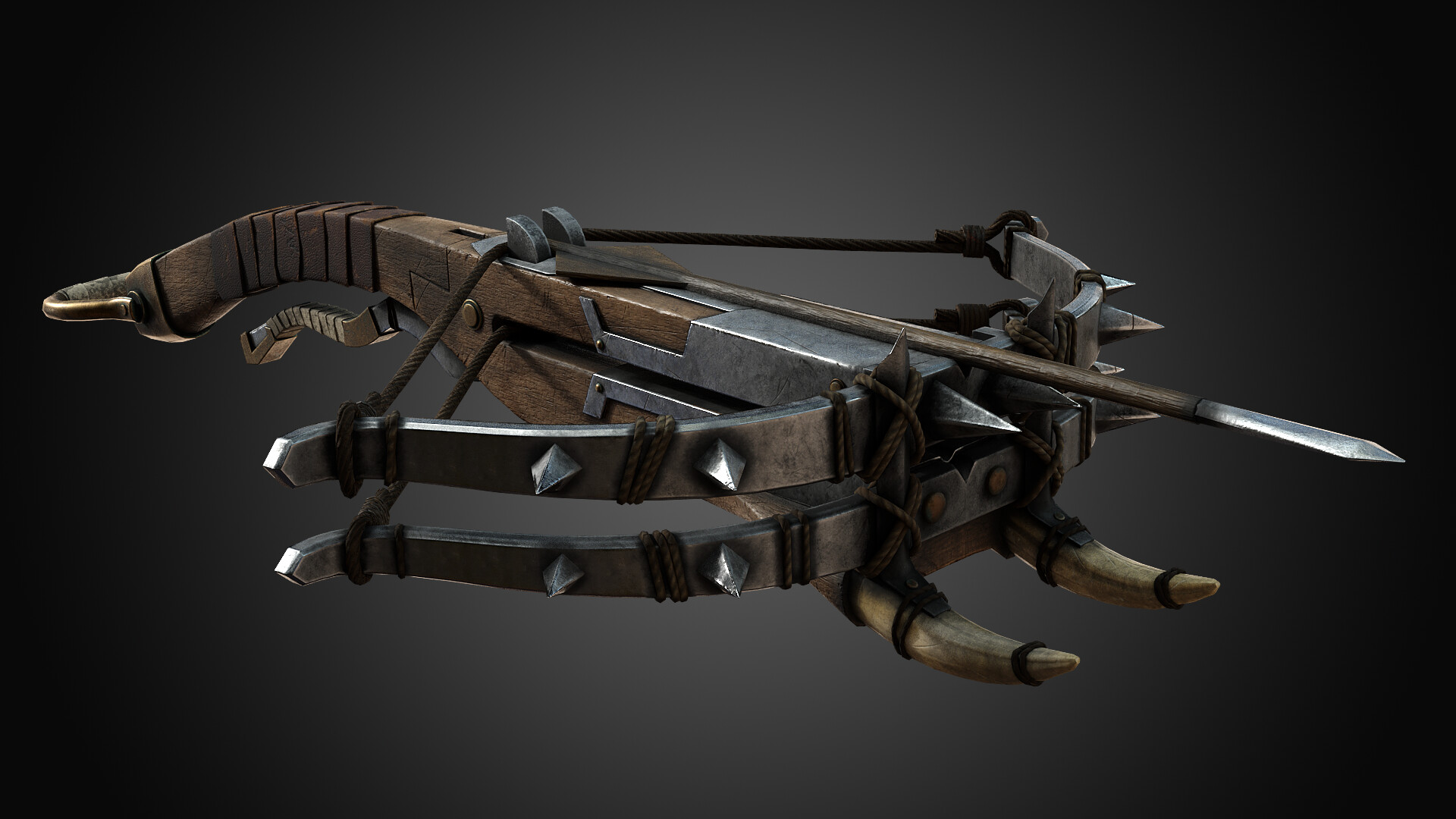This is a highly detailed, glossy, and professionally lit image of a medieval-looking crossbow, possibly computer-generated due to its unrealistic perfection. The crossbow is set on a shiny black surface, emphasizing its well-maintained condition which could suggest that it has been restored, potentially for a museum display. The crossbow is constructed from wood and iron, featuring two bows each adorned with little metal spikes, resembling fangs, likely to be used as additional weapons once the loaded arrow has been shot. The design includes sharp and pointy elements throughout, with a very sharp arrow already loaded into the shaft. The structure has intricate metal or steel accents, particularly around the end where the arrow is placed, and a trigger or cocking mechanism is evident under the back, enhancing its archaic yet formidable appearance.